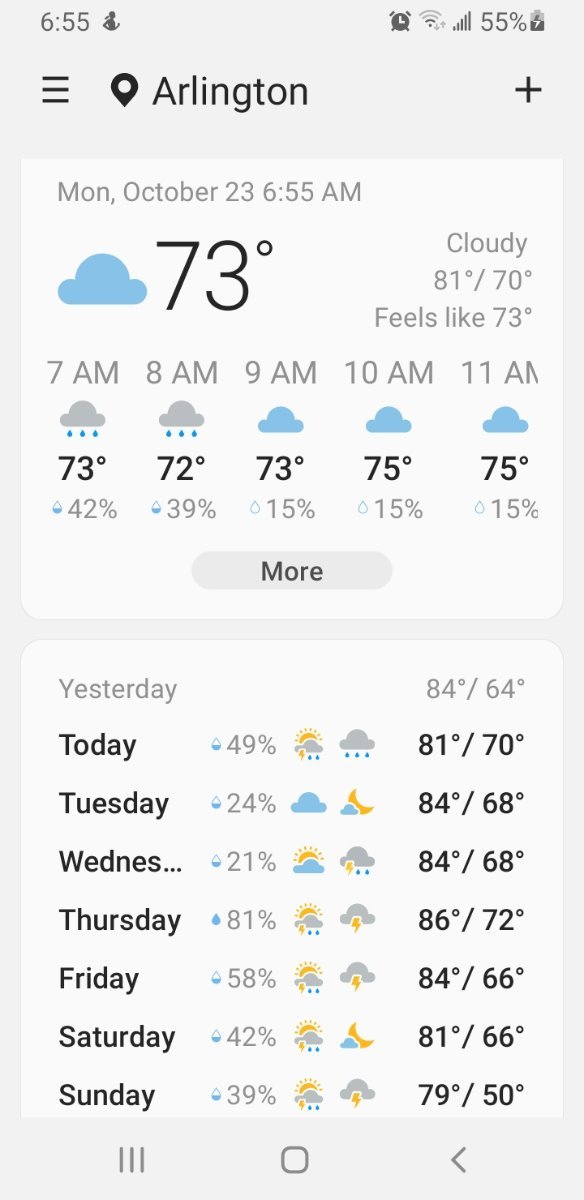The image displays a detailed weekly weather forecast for Arlington on a cell phone screen. At the top, there is a pin icon indicating the location, with "Arlington" labeled beside it along with a plus sign. Below this, the date is shown as Monday, October 23rd at 6:55 AM.

The current weather conditions are highlighted next: a blue cloud icon signifies that it is 73 degrees Fahrenheit and cloudy. The high for the day is 81 degrees, and the low is 70 degrees, with a "feels like" temperature of 73 degrees.

Further down, the hourly forecast for the morning is shown. At 7 AM, it is 73 degrees with a 42% chance of rain, indicated by a small rain cloud icon. At 8 AM, it is 72 degrees with a 39% chance of rain and a small rain cloud icon. At 9 AM, the temperature increases to 73 degrees with a 15% chance of rain and a blue cloud icon without rain. By 10 AM, the temperature climbs to 75 degrees with a 15% chance of rain and a blue cloud icon, which continues through 11 AM.

A button labeled "More" suggests access to additional information. Below, the screen summarizes the previous day's weather with a high of 84 degrees and a low of 64.

Today's weather is prominently displayed, with a 49% chance of rain, partly cloudy and rainy conditions, and high and low temperatures of 81 and 70 degrees, respectively, both in bold.

The upcoming week's forecast is detailed as follows:
- Tuesday: 24% chance of rain, partly cloudy in the evening, with a high of 84 degrees and a low of 68.
- Wednesday: 21% chance of rain, high of 84 degrees, and a low of 68.
- Thursday: 81% chance of rain with a high of 86 degrees and a low of 72.
- Friday: 58% chance of rain, with temperatures reaching a high of 84 degrees and a low of 66.
- Saturday: 42% chance of rain, high of 81 degrees, and a low of 66.
- Sunday: 39% chance of rain, with a high of 79 degrees and a low of 50.